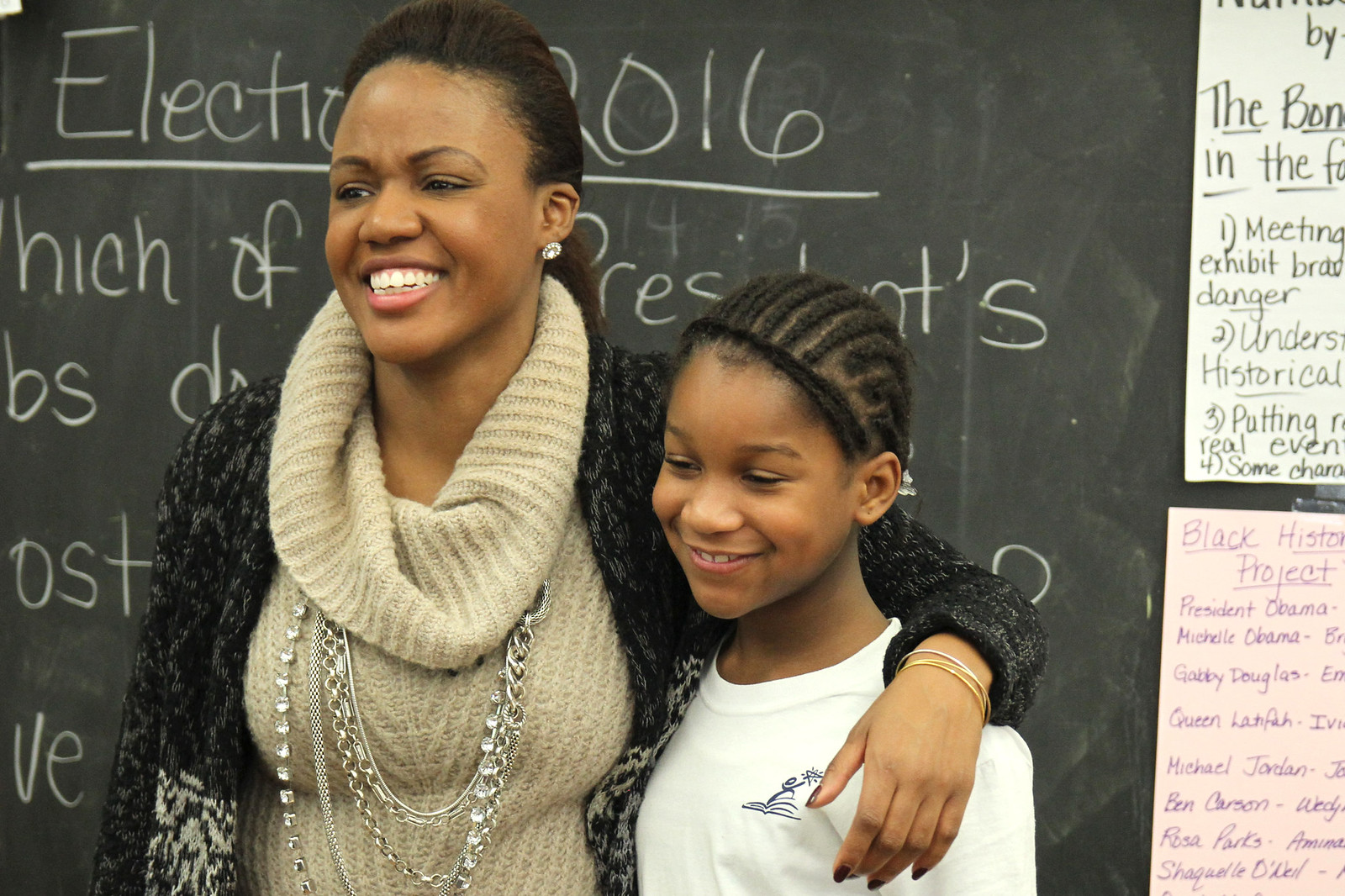This close-up photograph, taken indoors with excellent lighting, captures an African-American woman with her arm around a young African-American girl. They are positioned in front of a blackboard featuring educational content. The woman, resembling Michelle Obama, wears diamond earrings, multiple necklaces, a black and gray knitted cardigan over a tan sweater, and smiles warmly with her dark brown hair pulled back into a ponytail. The young girl, around 10 to 12 years old, has her hair styled in cornrows with braids forming a headband, and she is also smiling while wearing a white shirt.

The blackboard behind them displays text partially obscured by their presence but includes the phrases "Electrics 2016" or "Election 2016" and mentions presidents, possibly part of an educational discussion. Additionally, two pieces of paper are taped to the blackboard. The pink paper notably headlines a "Black History Project" that includes figures such as President Obama, Michelle Obama, Gabby Douglas, Queen Latifah, Michael Jordan, Ben Carson, Rosa Parks, and Shaquille O'Neal. Above, a partially visible white sheet contains phrases like "Meeting Exhibit Danger, Understanding Historical, Putting Real Even." This scene appears to be from a classroom, highlighting an educational and historical project.